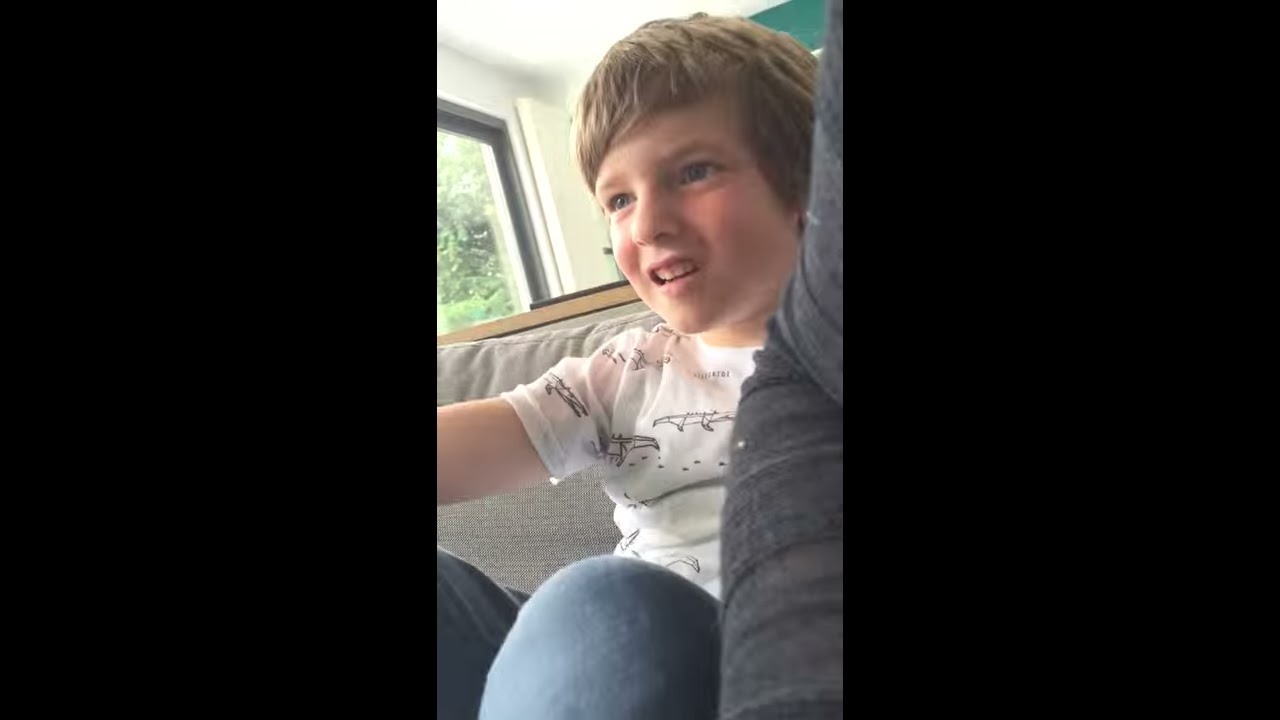In this image, a young boy with short dark brown hair is the focal point, sitting indoors, likely on a couch in a well-lit room with a window in the background. The boy, possibly around 8 or 9 years old, is dressed in a white short-sleeved t-shirt featuring an illustrated design that could be crocodiles or dinosaurs, and blue jeans. The boy's eyes are open, and his mouth is slightly ajar, exposing his top front teeth, suggesting he might be watching something with a hint of curiosity or confusion on his face. His knees are visible at the bottom of the image, indicating he is seated. The image is cropped in a portrait orientation and framed by black vertical rectangles on both the left and right sides, hinting that it might be a screenshot from a social media platform like TikTok, Instagram, or Facebook. Off-screen, another individual, partially visible and wearing dark clothing, is present beside the boy, turned away from him. The natural light streaming from the window indicates that it is daytime.